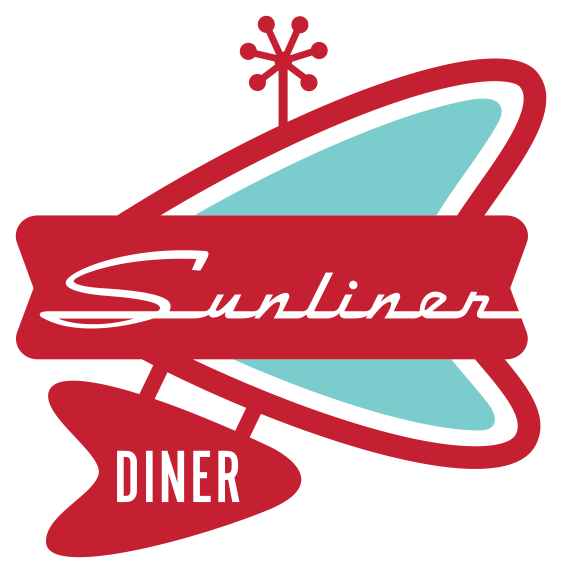The logo for the Sunliner Diner is a vintage, predominantly red design with nostalgic elements reminiscent of the 1950s or 1960s. The center of the logo features the name "Sunliner" in elegant white cursive text across a horizontal red strip. Below this, the word "Diner" is displayed in bold, white block letters within a red, arrow-shaped section resembling a guitar pick. The background is primarily white with a striking red border and a touch of blue near the top. At the top of the logo, a six-pointed pinwheel shape with round bulbs on each spike adds a whimsical, retro touch. The simplistic and clean design is suitable for web design or magazine advertising.